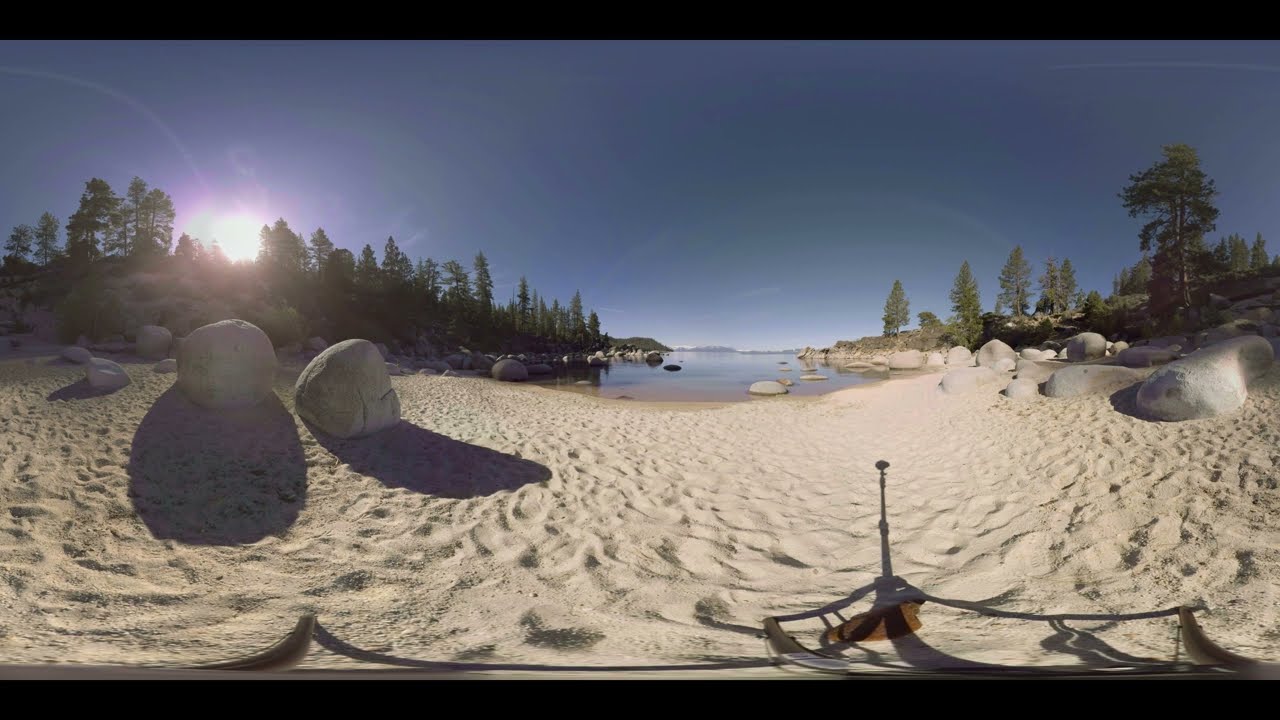The picture depicts a serene lakefront setting, possibly created using virtual reality due to its extremely high resolution and some noticeable warping. The scene features fine, light-colored sand that extends across the lower portion of the image, dotted with large boulders and rocks. The lake sits peacefully in the middle ground, flanked on both sides by rolling hills covered in tall, lush green trees. In addition to the trees framing both sides of the lake, the sky above is a dynamic mix of varying shades of blue with a notable purplish glow emanating from a setting sun located about a quarter of the way down from the top-left corner of the frame. Thin rectangular lines at the top and bottom of the picture suggest some framing technique, adding to the overall pristine and almost surreal quality of this landscape.